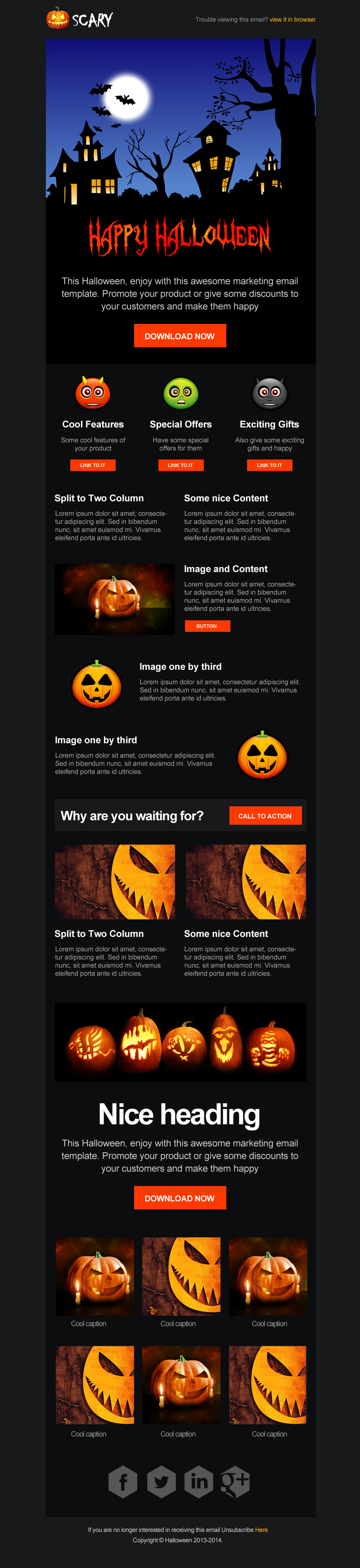This image is a long, vertical screenshot with a completely black background. At the top, there's the word "Scary" in white font accompanied by a small pumpkin icon to the left of the text. Below this, in bold orange letters, is the phrase "Happy Halloween". Above the text, a dark, cartoon-like night scene unfolds, featuring a moon shining down on a couple of black houses with orange-lit windows to signify that it is nighttime. Several bats can be seen flying around the moon, adding to the eerie ambiance. A barren tree, typical of October with no leaves, stands silhouetted in the scene.

Further down the image, there is an orange button with an unreadable white font on it, followed by three different selectable options represented by heads in colors orange, green, and dark gray. Each option is paired with an accompanying orange button underneath it.

Continuing down, a series of sections contain white text with a few sentences each. Towards the center, a pumpkin is placed on the left with corresponding white text on its right, and symmetrically, another pumpkin on the right has white text on its left. Moving downwards, there is a phrase in white text asking "what are you waiting for?" accompanied by an orange button to its right. Several more pumpkins are scattered below this section.

As we near the bottom, a prominent heading in white font is followed by another orange button. The image concludes with six more photographs of pumpkins arranged neatly at the bottom, each capturing the essence of Halloween.